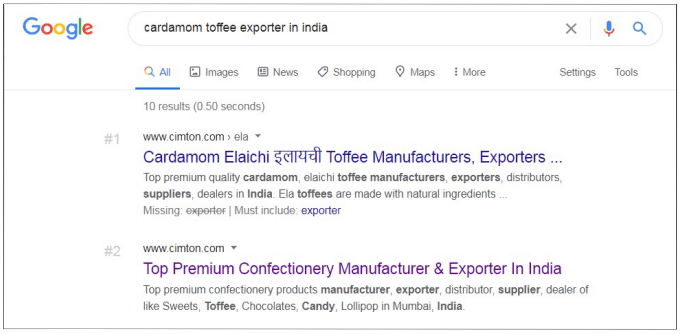A screenshot of a Google search page is displayed, showcasing a clean, white background. Positioned in the upper left corner is the iconic colorful Google logo, followed by the search bar that contains the query "cardamom toffee exporter in India." Underneath the search bar are various filter options, including "All," "Images," "News," "Shopping," "Maps," "More," "Settings," and "Tools." A thin gray line separates these options from the search results.

The search results indicate "About 10 results (0.50 seconds)" just above the first result. The first search result is marked with the number 1 and its URL is www.w.simpton.com. The clickable blue title reads, "Cardamom Elaichi Toffee Manufacturers Exporters," followed by a detailed description in black text: "Top premium quality cardamom elaichi toffee manufacturers, exporters, distributors, suppliers, dealers in India. Ela toffees are made with natural ingredients." The second result is marked with the number 2, although its details are not fully visible in this screenshot.